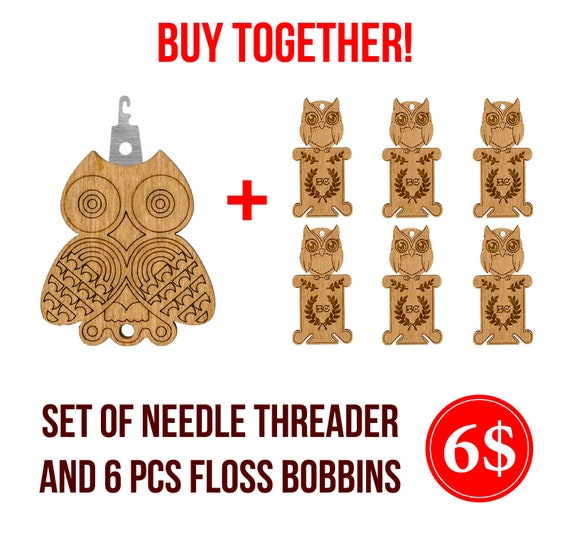The image on a solid white background prominently features the text "BUY TOGETHER!" in all caps red letters at the top. Below this, on the left side, is a detailed illustration of a wooden owl with large dark brown eyes, outstretched wings, and two feet. The owl has a metallic rectangular piece with a hook at the top attached to its head, suggesting it can be hung up, and it resembles a needle threader. Beneath it, there is a small hole cut out at the bottom.

To the right of the owl is a large red plus sign. Adjacent to this is a grid of six smaller owls arranged in two rows of three. Each of these smaller owls also has a hole at the top but none in the bottom and lacks the metal piece. These smaller owls are also light brown with dark brown eyes and have the letters "BC" on their bodies encircled by a leaf-like pattern.

In the lower left section of the image, in all caps brown letters, it reads "SET OF NEEDLE THREADER AND SIX PIECES FLOSS BOBBINS." The floss bobbins are what the smaller owl figures represent. Finally, in the lower right corner, there is a red circle displaying the price as "$6" with the dollar sign oddly placed after the number, creating a unique but slightly confusing presentation.